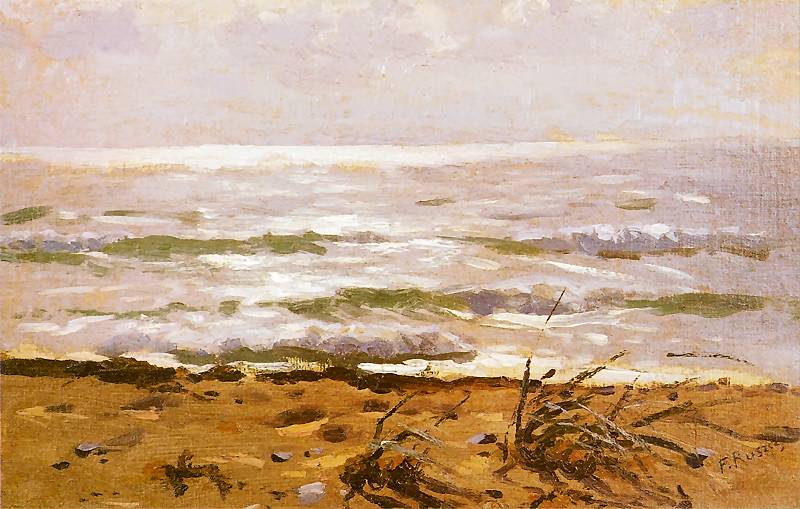This painting portrays a serene coastal scene divided into three distinct horizontal sections, each capturing different elements of the beach environment. The bottom third depicts a sandy beach with hues of light brown and tan, interspersed with streaks of yellow, likely representing the sunlit sand. The beach is dotted with small twigs, dead plants, and spiky, crab-like forms that lend an intriguing texture to the foreground. Scattered stones and rocks are also visible along the shoreline.

Transitioning to the middle third, the painting presents the ocean rendered in a semi-abstract, impressionistic style. The water exhibits a blend of colors, including bright and light oranges, pinks, whites, and varying shades of green and gray, suggesting a dynamic interplay of sunlight and waves. The impressionistic waves convey a sense of movement and reflect a bright, sunny day.

In the top third, the sky spans with a pale gray tone, subtly infused with touches of yellow and white, depicting faint clouds, particularly visible on the left side. This part of the painting conveys a calm yet slightly overcast atmosphere. The horizon is marked by a delicate yellow line, enhancing the ethereal quality of the scene.

The painting is signed "F.R.U.S.Z.I.G." at the bottom, adding a personal touch to this evocative portrayal of a tranquil beach.